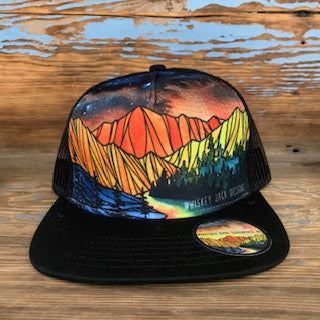This image features a black baseball cap with a flat brim, positioned squarely in the center of the frame. The hat is situated on a rustic, weathered wooden surface that resembles a picnic table, characterized by visible cracks and patches of worn greenish-blue paint. In the background, there's a wooden wall with additional blotches of blue paint.

The front of the cap showcases a vivid and detailed illustration. This artwork includes a series of red, yellow, and orange mountains, with a prominent canyon-like appearance. At the lower right of the image on the cap, the word "Whiskey" is discernible. Below the mountains, there is a flowing river depicted in rainbow colors, flanked by pine trees and rocky terrains at the lower left. The upper part of the cap design features a night sky teeming with stars and accented by a hint of pink, evoking a sense of a cosmic or space theme.

Additionally, the cap's brim bears a sticker replicating the same intricate mountain and river scene found on the front of the hat. This sticker is situated on the right side of the brim, incorporating similar vivid colors such as yellow, orange, blue, and purple. Together, these elements form a cohesive and visually striking depiction on both the cap and sticker, emphasizing the natural and celestial motifs intertwined in the design.